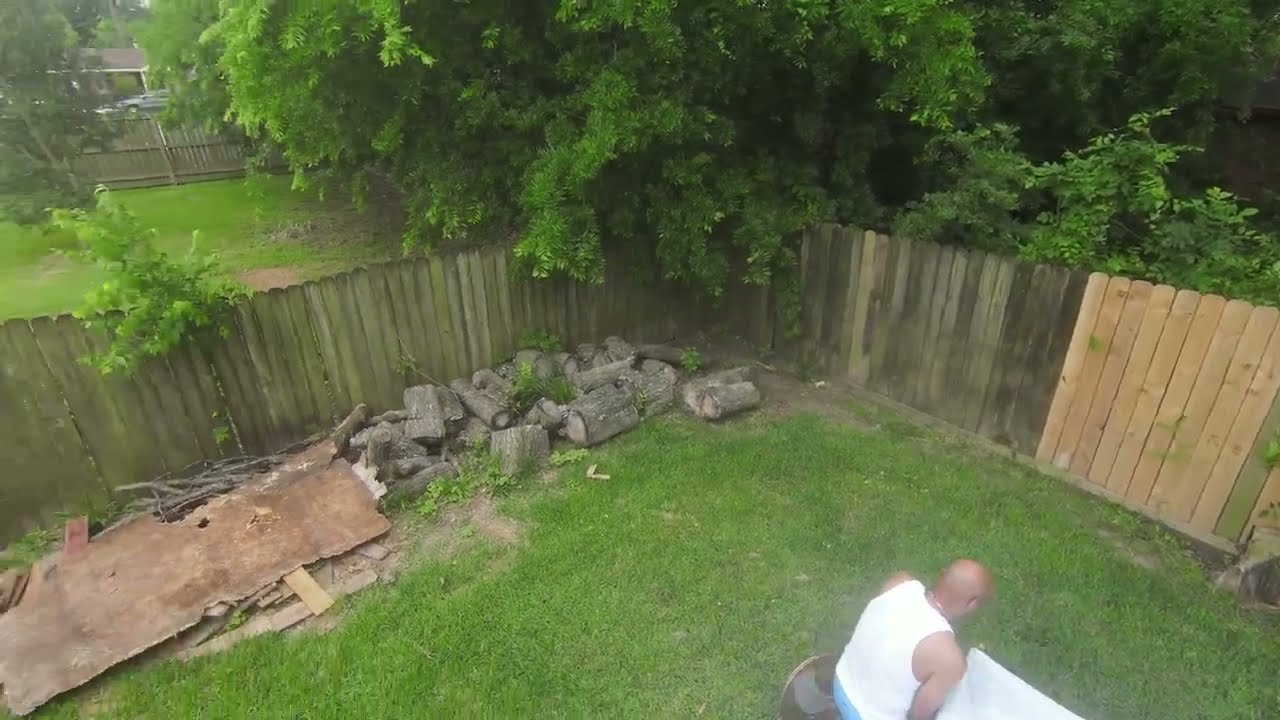Aerially viewed, this image captures a backyard scene featuring a bald, black man dressed in a white tank top and blue shorts, possibly accessorized with a gold chain. This man, positioned in the bottom right corner, leans forward, perhaps examining the slightly overgrown green grass beneath him. Adjacent to his right is a small white piece of cloth. The rectangular yard is delineated by a wooden plank fence; the planks on the right appear newer than the weather-beaten, gray and greenish planks forming the rest of the enclosure. Chopped logs are scattered in the upper left corner, near a large sheet of metal. To the left, suggesting ongoing work, lie several concrete blocks and uprooted materials. Beyond the fence, a dark, leafy tree casts a shadow, and neighboring yards with similar fencing and green grass stretch out, revealing a carport and partial view of a parked car in the upper left corner.